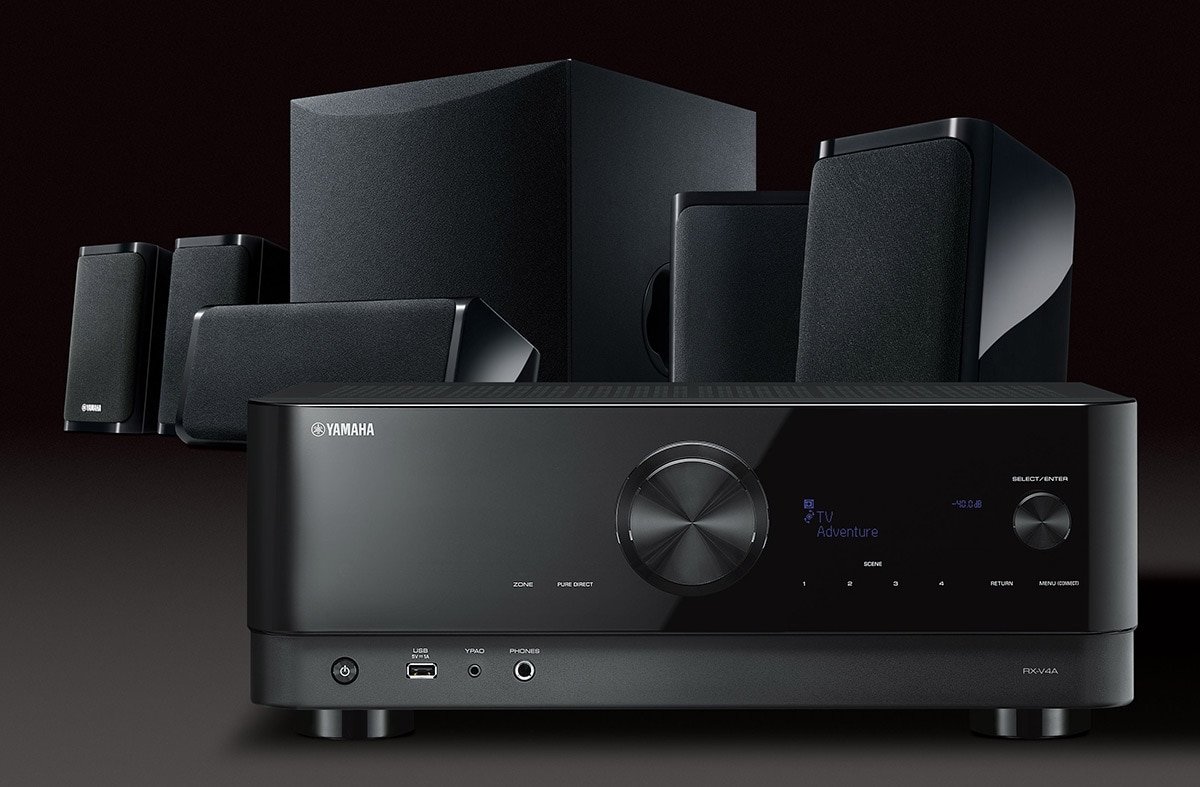Here we have a highly professional studio photograph showcasing a Yamaha surround sound system. The central piece is a sleek, black, rectangular Yamaha device with a rounded facade, prominently featuring two circular knobs—one large knob centrally placed and a smaller knob to the right. At the top left of the device, "Yamaha" is displayed in white letters, and there are additional blue letters spelling "TV Adventure." At the bottom of the device, you can find a few ports and a power button. 

Behind the main device, there are six black audio speakers arranged in a symmetrical pattern. Four standing speakers of identical size are positioned symmetrically along the sides. In the middle, a horizontally oriented speaker lies in front of a larger, square-shaped subwoofer. The entire setup exudes a professional ambiance, enhanced by the black background that adds a sophisticated, monochromatic elegance to the image.